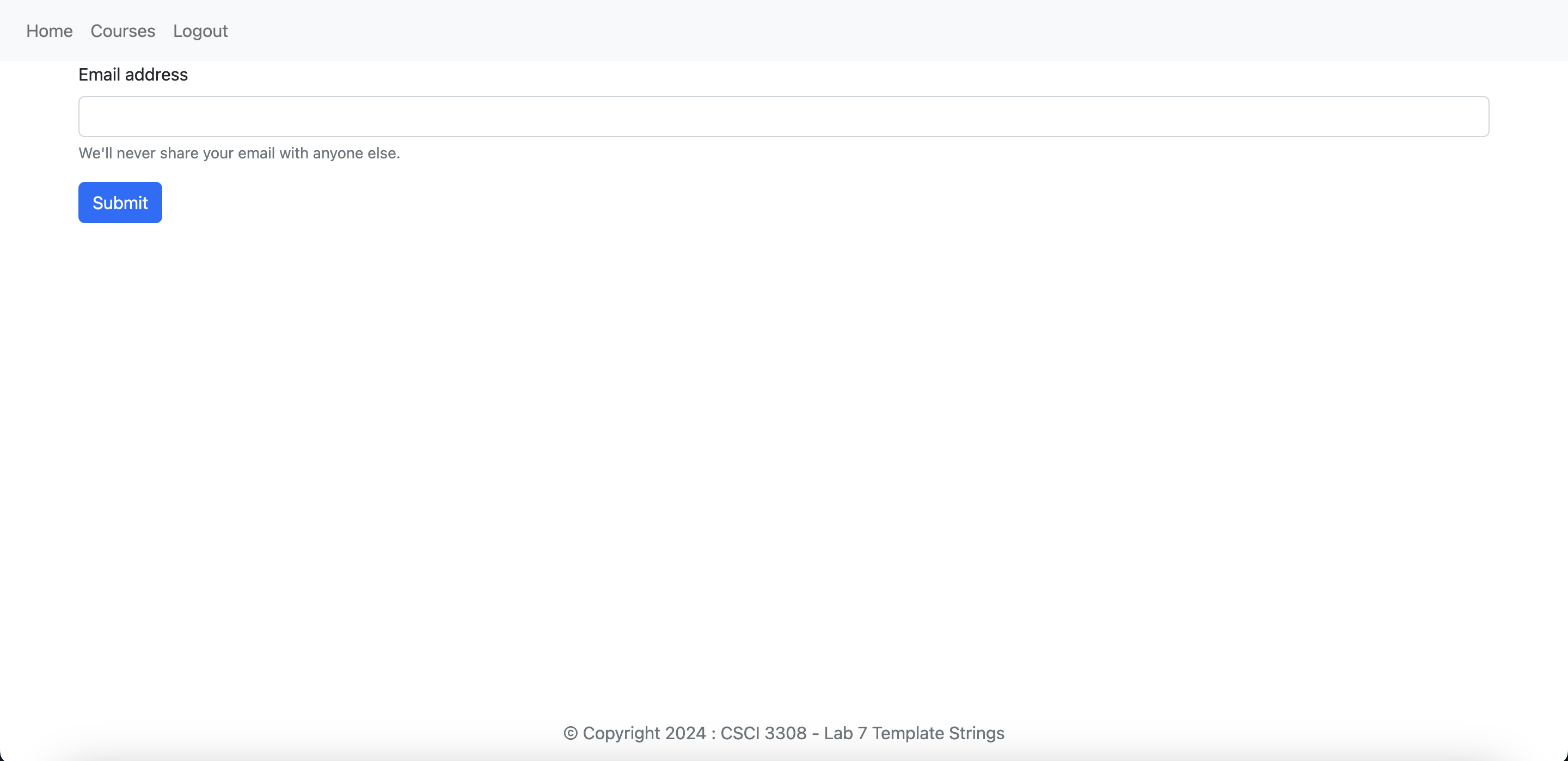This image is primarily a minimalistic user interface for what appears to be an online course login page. Dominating the upper left-hand corner of the page are three navigation links labeled "Home," "Courses," and "Logout." Below these options, there is a placeholder prompt for an "Email Address" with a rectangular text entry field ready for input. Directly underneath the input field is a privacy assurance statement that reads, "We will never share your email with anyone else." Further down, there is a prominent blue "Submit" button designed for users to click after entering their email address. At the very top of the page, small text reads, "Copyright 2024, CSCI 3308-LAB7, Template, Strings." The rest of the page appears largely blank or pale, possibly as a design choice. A subtle arrow at the bottom may either be a part of the interface or simply a spot on the screen, adding a hint of imperfection to an otherwise sparse and clean design.